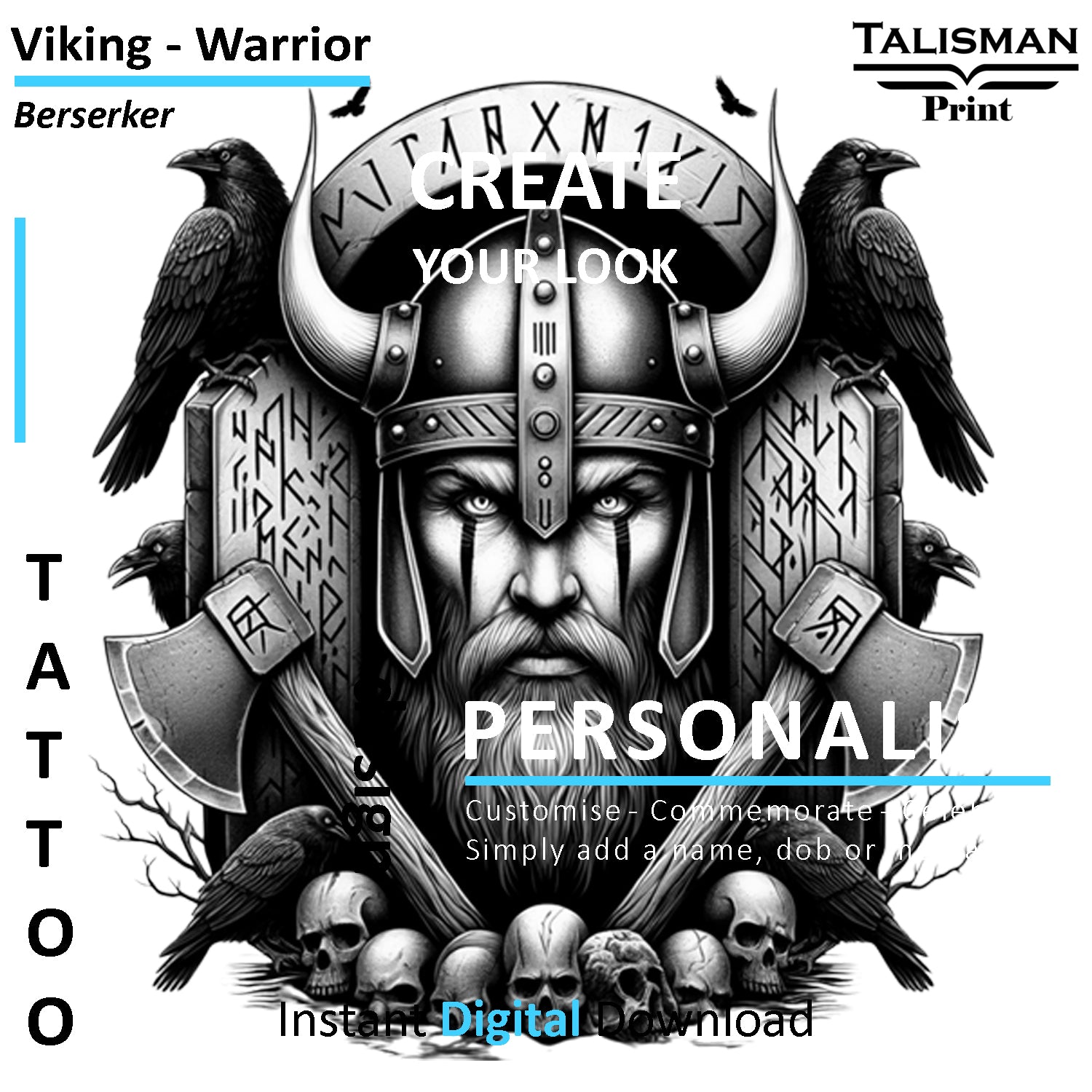This image is a detailed drawing that appears to be an advertisement for a personalized digital download featuring a Viking theme. In the top left corner, it reads "Viking Dash Warrior," underlined in light blue. Below that, in black letters, it says "Berserker," accompanied by a vertical light blue line with the word "Tattoo" written vertically in black. The top right corner displays "Talisman Print." 

Central to the image is the head of a Viking warrior adorned with horns, bearing a beard, mustache, and face paint under the eyes. Two black crows flank his head, perched next to rune-engraved tablets. Additionally, two axes with their handles embedded in the ground form a V-shape beneath his chin, surrounded by a pile of human skulls. Above the Viking's helmet, rune script arcs between the horns, with the words "Create Your Look" displayed at the top.

The middle section invites users to "Personalize, Customize, Commemorate" by adding a name, date of birth, or other inscriptions. At the bottom, it mentions "Instant Digital Download." The overall image gives an impression of an avatar interface for a video game or a similar customizable avatar game setup.